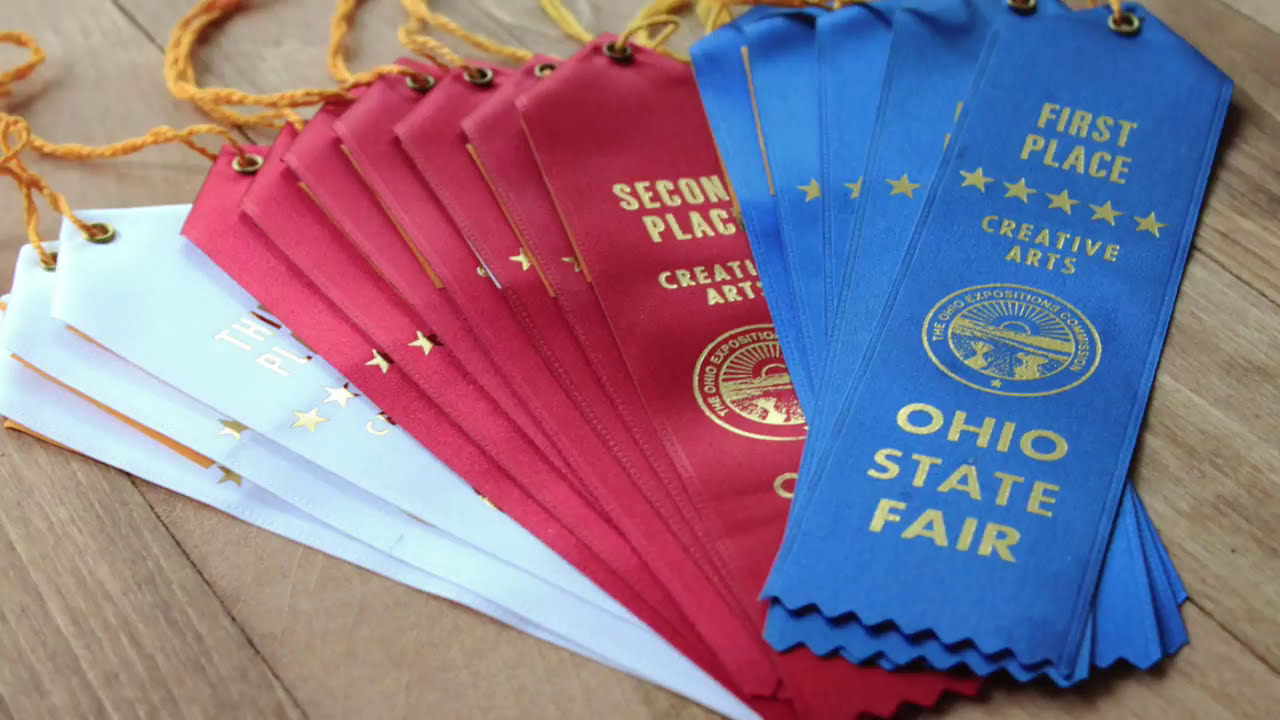The photograph showcases a detailed close-up of a collection of award ribbons from the Ohio State Fair, neatly fanned out on a light tan, unfinished wooden surface. The arrangement features three distinct sets of ribbons: at the bottom, white ribbons signifying third place, followed by a middle layer of red ribbons representing second place, and at the top, blue ribbons denoting first place. Each ribbon is adorned with gold lettering. The text on the blue ribbons reads "First Place, Creative Arts," followed by the logo of the Ohio Exposition Commission and "Ohio State Fair" in bold letters. This text and design are presumed to be the same across all ribbons, with appropriate variations in place designation. The ribbons feature goldish strings at the top, likely for hanging. The image is tightly framed on the ribbons, emphasizing their arrangement and the intricate details of the text, capturing the prizes' essence for creative arts competitions at the Ohio State Fair.